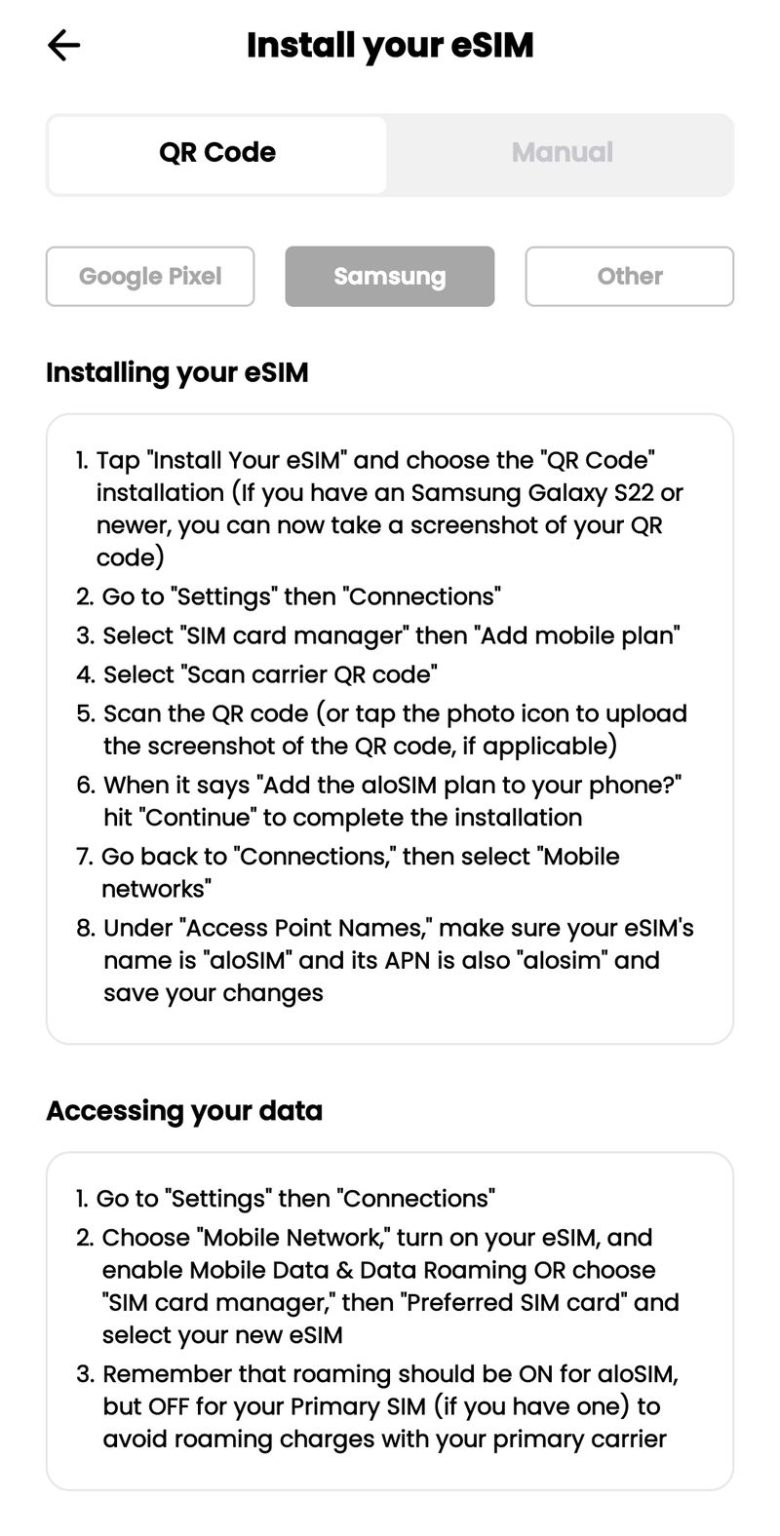This is a detailed screenshot from a cell phone, configured in a portrait orientation with a predominantly white background. In the top left corner, there is a black back arrow pointing left. Centrally, the text "Install your eSIM" is displayed prominently in bold black font, with "eSIM" fully capitalized. 

Below this, on the left side, there is a white rectangle covering about half the width of the screen. It contains the bold text "QR code." Adjacent to it on the right is a light gray tab labeled "Manual" in black text. Further down, in the center, there is a gray tab with the word "Samsung" inscribed in white. Flanking it on the left is a white tab with a gray border labeled "Google Pixel," and to its right, another white tab with a gray border labeled "Other."

Under these tabs, on the left side, is a section titled "Installing your eSIM," followed by a large square containing step-by-step instructions. Numbered 1 through 8 down the left margin, each step is accompanied by lines of detailed instructional text, varying from a single line to multiple lines of information.

Towards the bottom left, there is a bold section header "Assessing your data." Beneath this header, a line extends across and then down into a small rectangle. Inside this rectangle, on the left, is the number "1" followed by a sentence. Directly below, the number "2" precedes four lines of text. Finally, the number "3" is accompanied by three lines of information detailing data assessment processes.